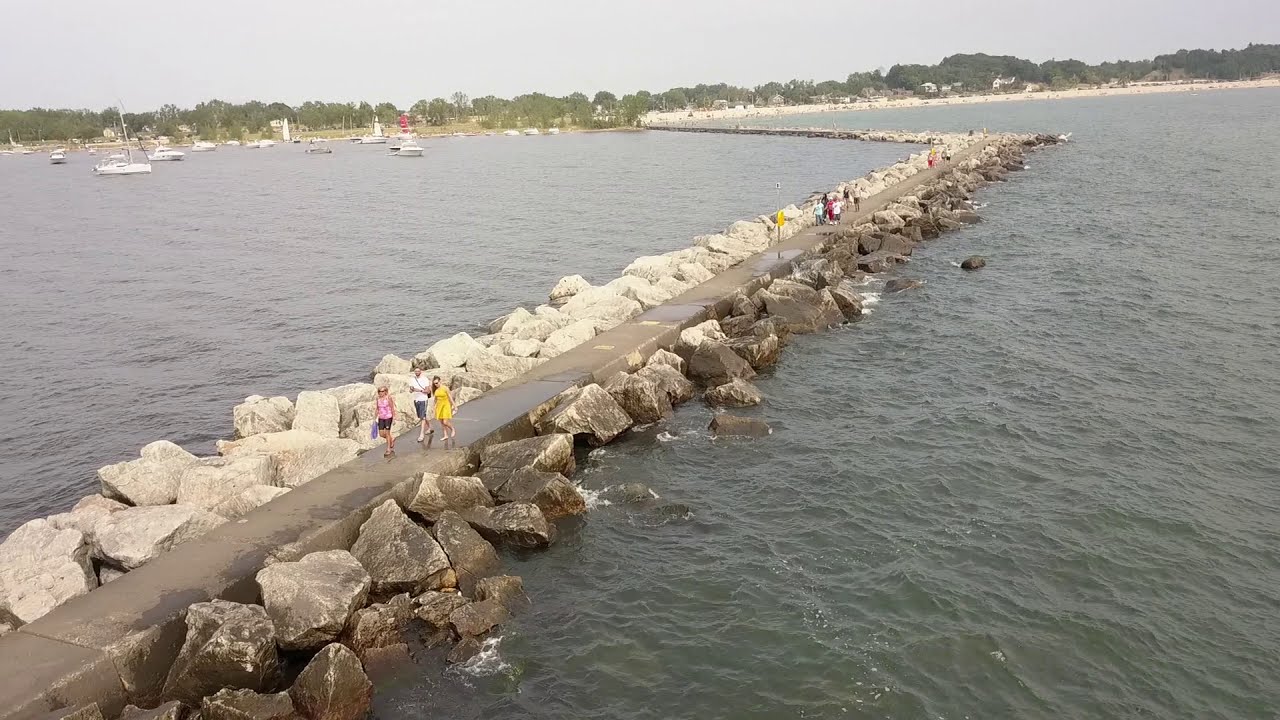The image depicts a narrow concrete walkway stretching across a calm body of water, forming an angled path supported by large, jagged rocks. Along this scenic trail, several people, including individuals in a pink shirt, white shirt, and yellow dress, are leisurely strolling. In the background, a serene bay is dotted with anchored sailboats, highlighting a tranquil marine setting. To the left, a prominent red lighthouse stands as a notable landmark. The horizon showcases a line of trees, merging with a clear sky above, under subtly overcast conditions, which cast a gentle, muted light across the scene. The setting evokes the tranquil coastal landscapes similar to those found in Michigan, possibly around Escanaba.